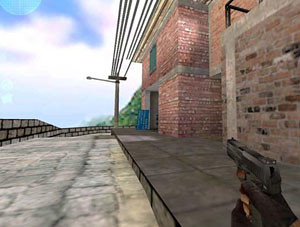This is a detailed screenshot from an early 2000s video game, potentially Counter-Strike or Half-Life, depicting a first-person view in a realistic outdoor scene. The player is holding a handgun, with visible fingers under black gloves, and is standing on a cobblestone road adjacent to a brick patio and brick buildings. The scene includes a sidewalk running alongside the road, a blue barrel next to a doorway on a brown building, and a stone wall across the street. Overhead, there are power lines and the blue sky adorned with some white clouds. In the distance, there's a hill covered in greenery and a streetlight is visible further down the road. The overall perspective creates an immersive atmosphere, characteristic of early 2000s video game graphics.